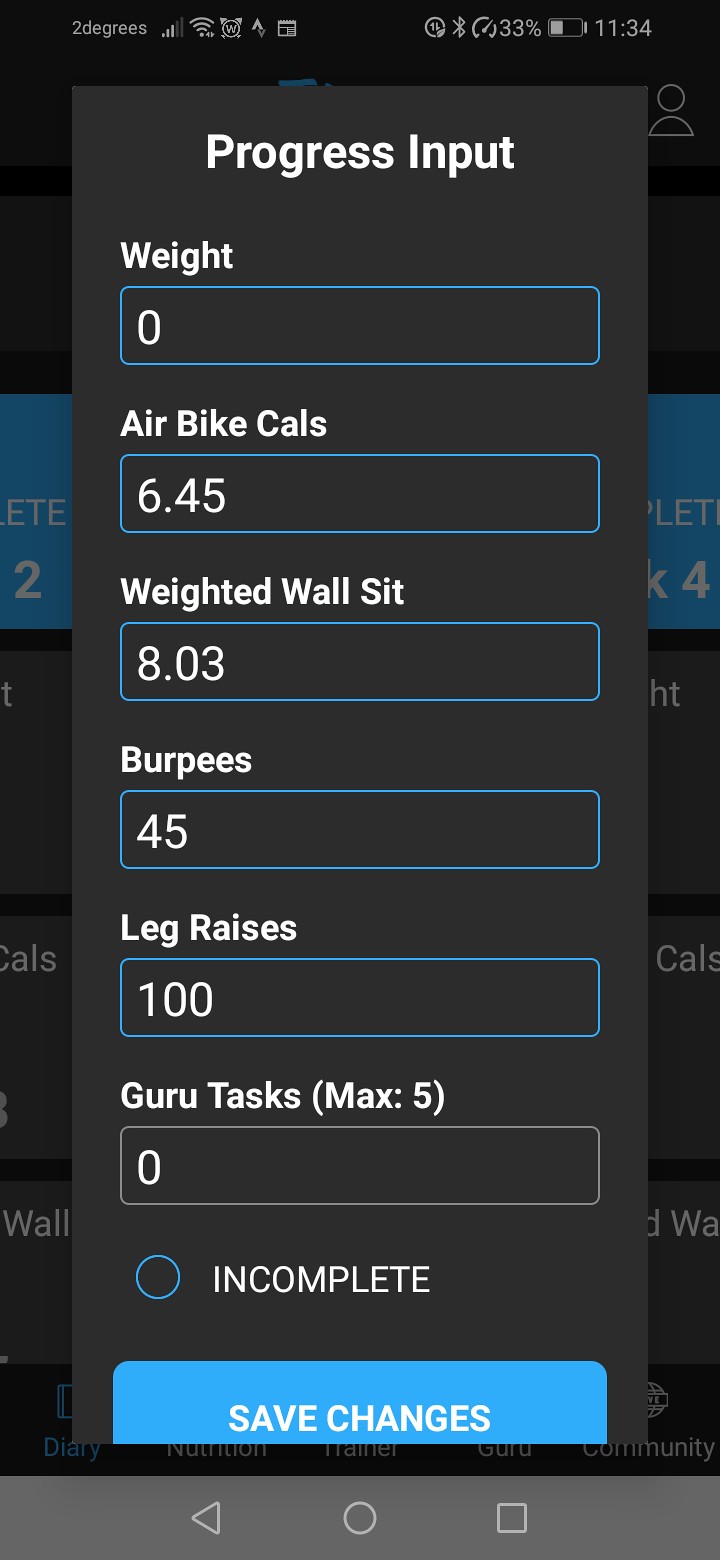The image is a detailed screenshot of a cell phone, featuring a workout app interface labeled "PROGRESS INPUT" in white text on a gray background. At the top, standard cell phone indicators display the current temperature, an active alarm, Bluetooth connectivity, 33% battery life, and the time, 11:34. Centrally, the app presents several fields for entering workout data:

1. **WEIGHT**: Currently set to 0.
2. **AIRBIKE CALS**: Displaying 6.45.
3. **WEIGHTED WALL SIT**: Showing 8.03.
4. **BURPEES**: Numbered at 45.
5. **LEG RAISES**: Marked at 100.
6. **GURU TASKS MAX 5**: Set to 0.

Below these fields is a prominent blue button labeled "Save Changes." Additionally, the bottom of the phone screen features a typical navigation bar with a triangle, circle, and square icons. The app interface, with its organized layout, clearly aims to track and save workout progress efficiently.